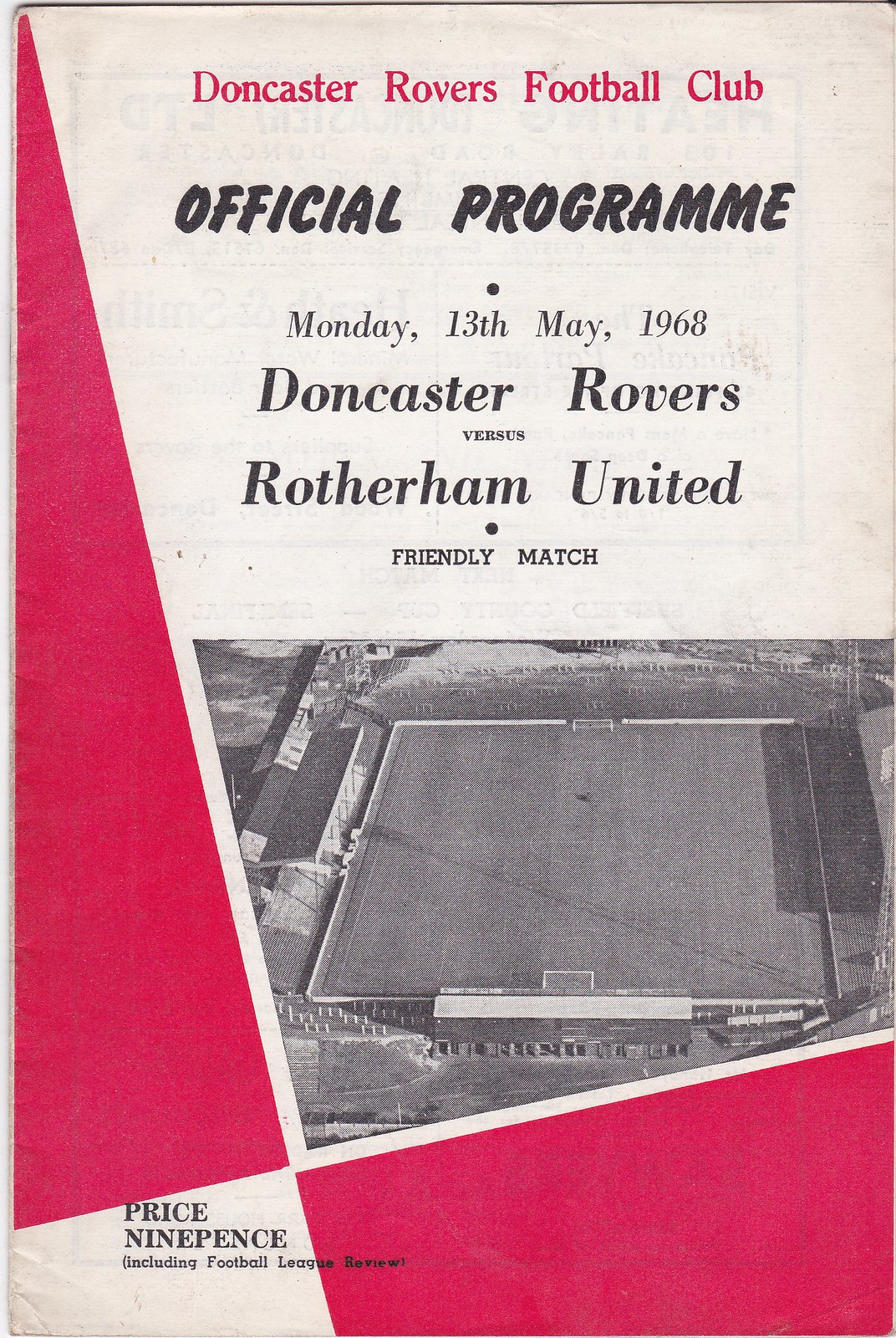The cover of the Doncaster Rovers Football Club official program dated Monday, 13th May, 1968, features prominently in red and black letters at the top. Below this, the names "Doncaster Rovers" and "Rotherham United" are highlighted, marking it as a friendly match. Central to the design is a black and white photograph of a football field, depicting goals at both ends, sidelines, and visible stands on the left. The image has a slightly grainy quality. A pink triangle decorates the left-hand side, extending from the top corner down to near the bottom, and there's additional pink shading in the bottom left corner. The bottom of the program displays the text "Price 9 pence, including Football League Review" in black writing on a white background.